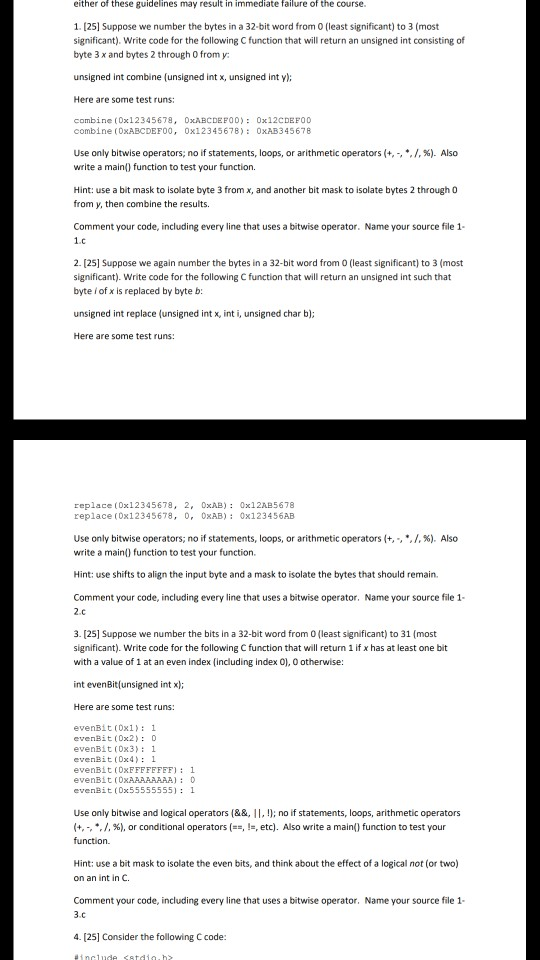Displayed is an image showing the bottom half of one page and the top half of another, separated by a pronounced black border that divides them both vertically along the sides and horizontally between the two pages. The text throughout the image is too small to read clearly. 

On the top page, the layout consists of several short paragraphs; many are single lines, separated by double or triple spacing. A few paragraphs extend to three lines each, and amid these sections, there appears to be a line that is in all capital letters.

The bottom page continues with a similar format but starts less densely, displaying two lines in a lighter, less bold font at the top, which seemingly represent numbers. About halfway down the bottom page, there is a section comprising approximately eight lines, which also seem to be composed of numbers or symbols.